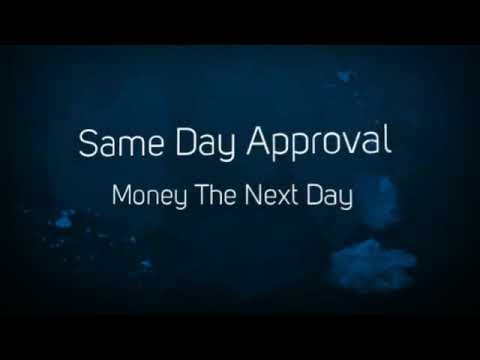The square image appears to be a still from a digital advertisement. It features prominent horizontal black borders at the top and bottom. The central section of the image has a dark indigo blue background, slightly blurred, interspersed with lighter blue and white splotches that give an impression of being underwater or depicting a fluid scene. There are gray rock-like formations visible off to the side, adding to the uncertain but aquatic feel. Centered in the image, bold white text reads "Same Day Approval" with a slightly smaller line of white text below it stating "Money the Next Day." Both lines of text are neatly aligned in the center.